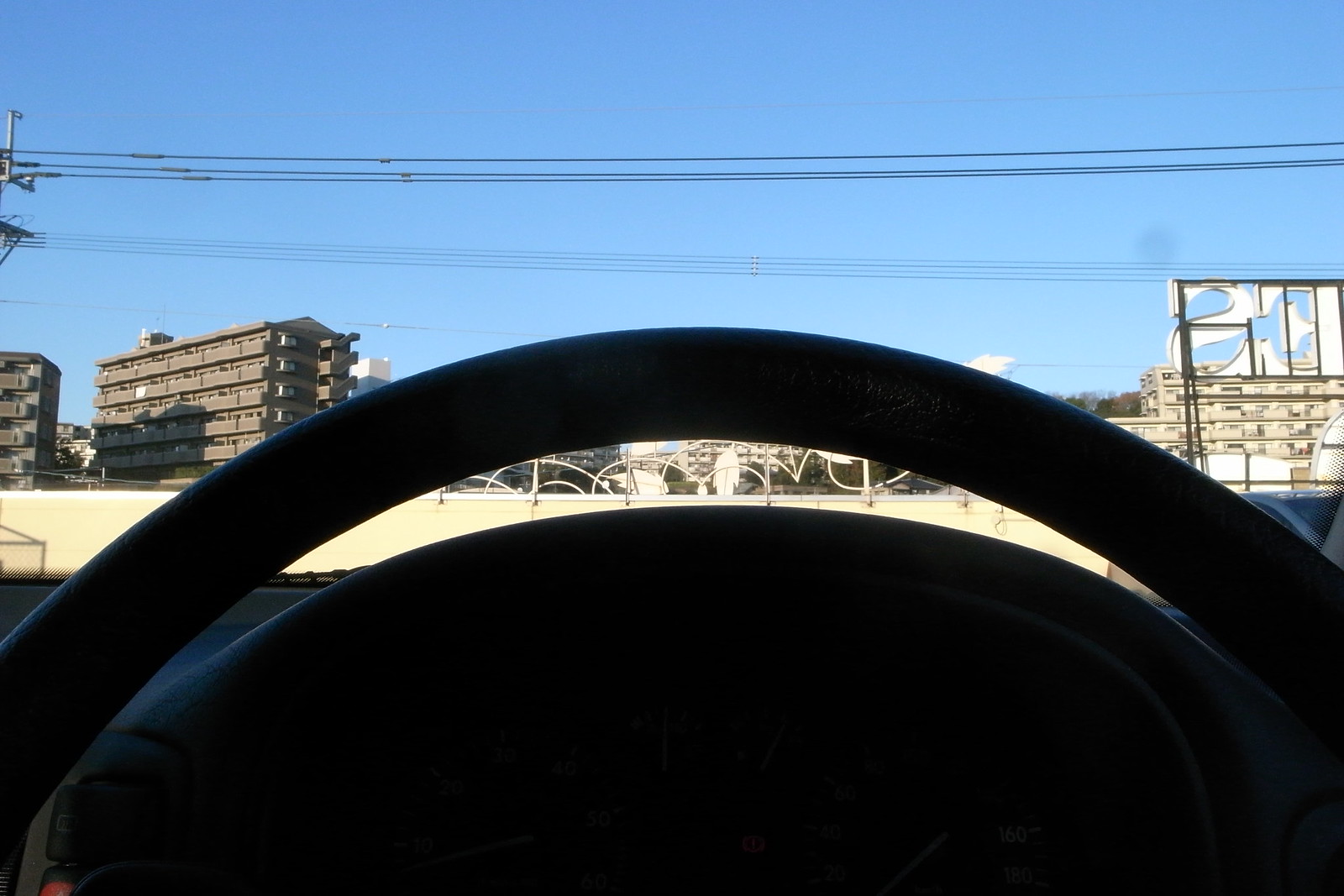Under a vivid blue sky devoid of clouds, horizontally aligned power lines stretch across the image, juxtaposing a cityscape featuring several large buildings. These structures, which appear to be hotels, dominate the scene with their imposing presence. On the right side, a partially visible sign affixed to one of the hotels displays the letters 'E' and 'S', though the full text is obscured. In the foreground, a dark, wheel-like object resembling a car steering wheel adds an intriguing element, though its exact nature remains ambiguous due to the small gap between the wheel and its connecting piece.